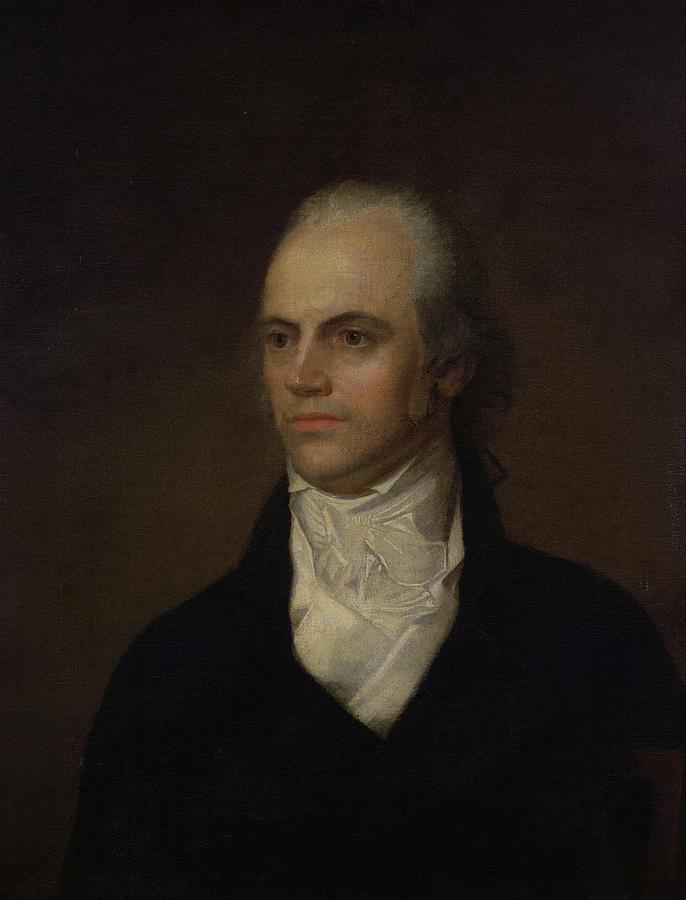This is a detailed painting, reminiscent of a 17th or 18th-century portrait, depicting a pensive white man with pronounced facial features. He wears a high-collared white shirt beneath a black coat that meets in the middle without any visible buttons, giving an impression of elegance with minimal detail in the fabric rendering. His face, framed by long, grayish hair that recedes at the hairline and potentially tied back, shows large brooding brown eyes and pronounced sideburns. The man also sports a slight five o'clock shadow, adding a touch of ruggedness to his otherwise serene and contemplative demeanor. He gazes slightly to the right, into the distance, creating a sense of introspection. The background transitions from dark hues to lighter shades around his face, enhancing the focus on his expressive eyes and thoughtful expression.